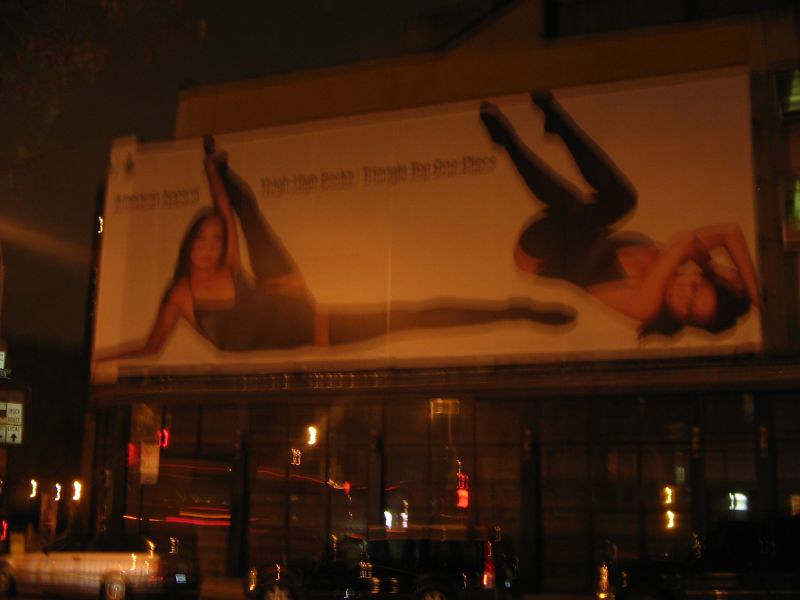In this nighttime photograph taken within a city or town, a prominent billboard dominates the scene. The image is somewhat blurry, adding a sense of atmospheric mystery, but the main elements remain discernible. The billboard showcases an advertisement featuring two women in elegant black lingerie. 

In the lower part of the image, street lights cast a soft glow on the scene, illuminating a row of parked cars with their shiny silver rims – notably, a white car and a black car. Above these vehicles, the billboard captures the eye. One woman, with dark hair, lies down with her knees raised, her hands positioned above her head. She is clad in a black negligee that exudes sophistication. To her left, the second woman strikes a graceful pose, lifting one leg high in the air and holding it with her left hand, while supporting herself with her right arm. She mirrors the first woman's attire, wearing similar black stockings and lingerie.

Accompanying the visuals, the text on the billboard hints at the nature of the advertisement: phrases like "thigh high socks" and "one piece" suggest that it promotes the lingerie being worn by the models. Through this detailed and evocative nighttime scene, the billboard effectively captures both attention and allure, highlighting the elegance of the products being advertised.